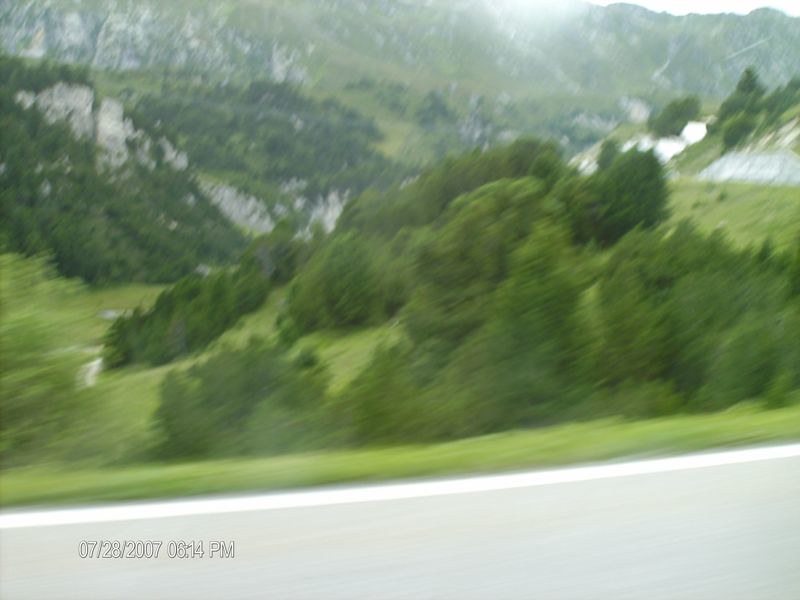A photograph dated July 28, 2007, at 6:14 PM captures a serene landscape. The bottom edge of the image offers a brief view of a road, above which stretches a verdant expanse of trees. The foliage displays a spectrum of colors, from deep green to a paler, almost white shade, with subtle touches of faint yellow interspersed among the leaves. The background features impressive rock formations, blanketed with dense tree cover and patches of moss. Above the rocky outcrops, a gentle sunlight filters through, casting a natural luminance across the scene. The rocks themselves exhibit hues of gray, off-white, and brown, adding to the rich texture of the rugged landscape. The image, slightly blurred, captures the tranquil ambiance of a lush, natural setting.